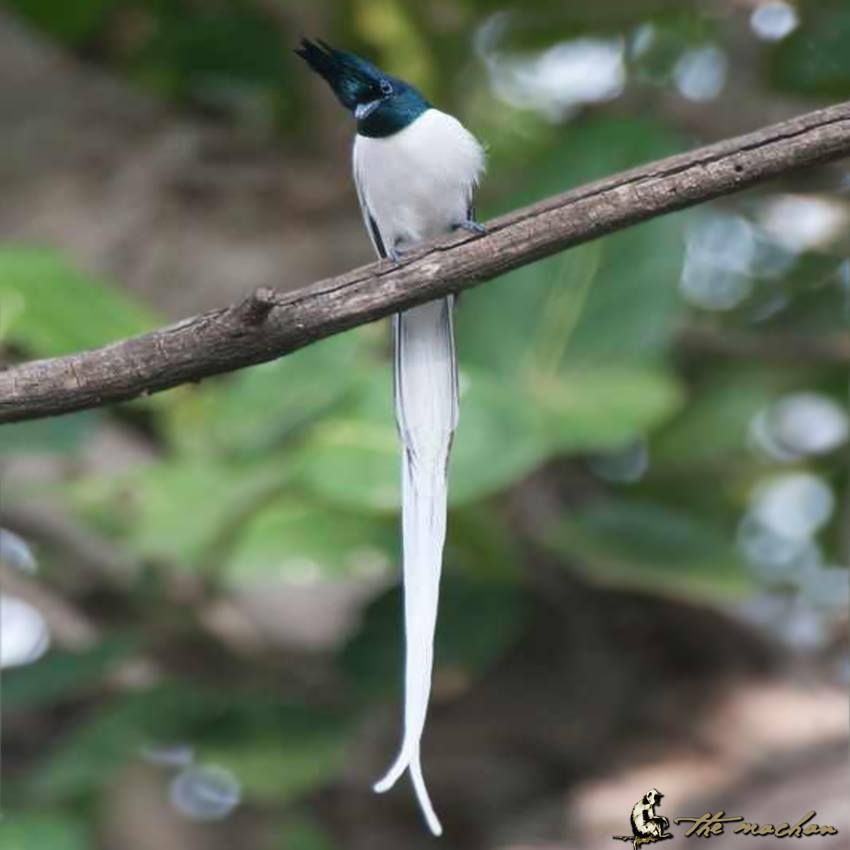The image captures a striking and possibly rare bird perched on a thin, light brown tree branch that stretches across the entire frame. The bird, mainly white with contrasting dark indigo (or black) head feathers, features a distinctive mohawk. Its long, elegant white tail spans nearly twice or even three times the length of its body, ending in two prongs, and dominates over half of the photo's height. The bird is looking curiously at the camera, its head turned slightly 45 degrees to the right. The blurred background suggests a rainforest or wooded environment filled with leaves and branches, adding depth to the photograph. In the lower right-hand corner, a small logo of a monkey sitting on a branch with cursive text spelling "Mashon" or "Mekang" is visible. The bird's intense eyes and sleek beak contribute to its captivating presence in this detailed and vivid snapshot.